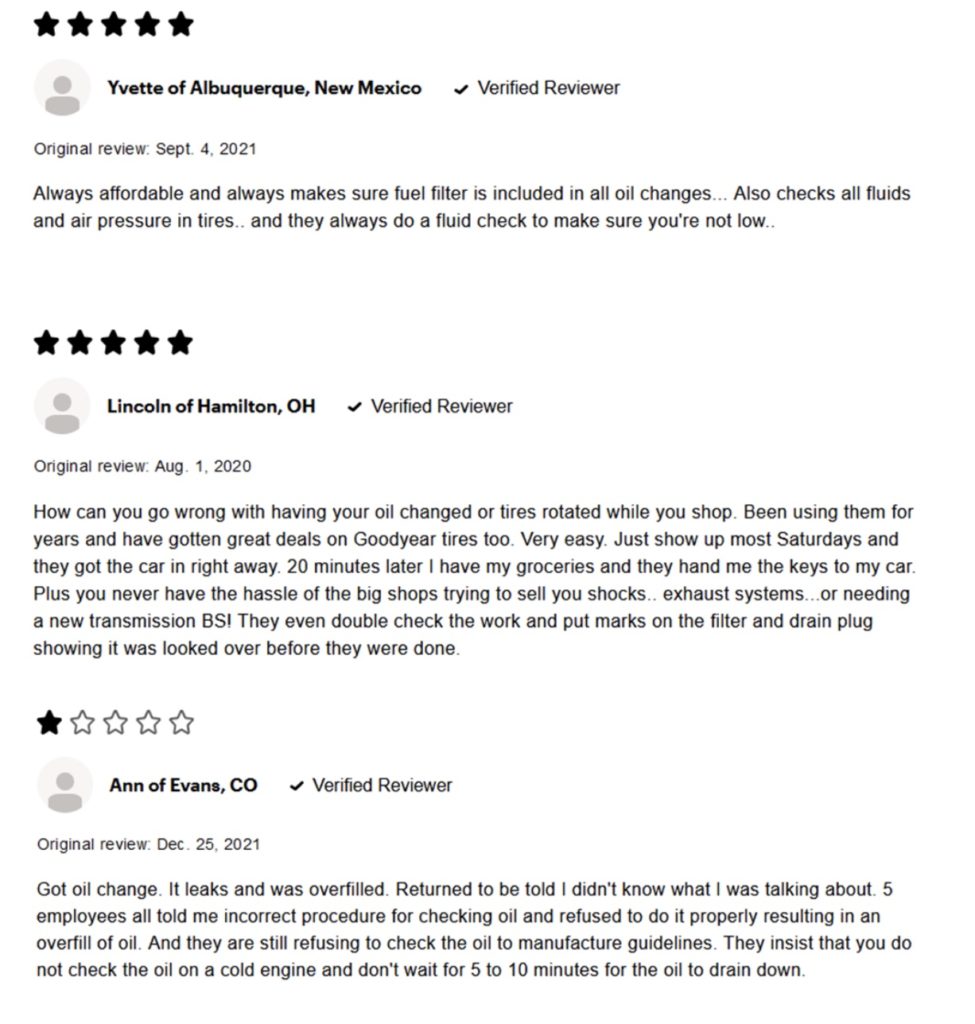The image is a screenshot of a review website showcasing three distinct reviews for an auto repair shop. The website prominently features a star rating system, with the bar of stars highlighted in black, making them impossible to miss.

The first review boasts a five-star rating attributed to Yvette from Albuquerque, New Mexico. Yvette is marked as a "Verified Reviewer," lending credibility to her feedback. Her review is concise and straightforward: "Always affordable, always make sure fuel filter is included in all oil changes." 

The second five-star review comes from Lincoln in Hamilton, Ohio, who is also a "Verified Reviewer." Lincoln provides a more detailed account of his positive experiences with the auto repair shop, commending the various services he received.

Contrasting the positive feedback, the third review is a one-star rating given by Ann from Evans, Colorado. As a "Verified Reviewer," Ann's negative experience carries weight. She expresses significant dissatisfaction and outlines the issues she encountered during her visit, delivering a harsh critique of the establishment.